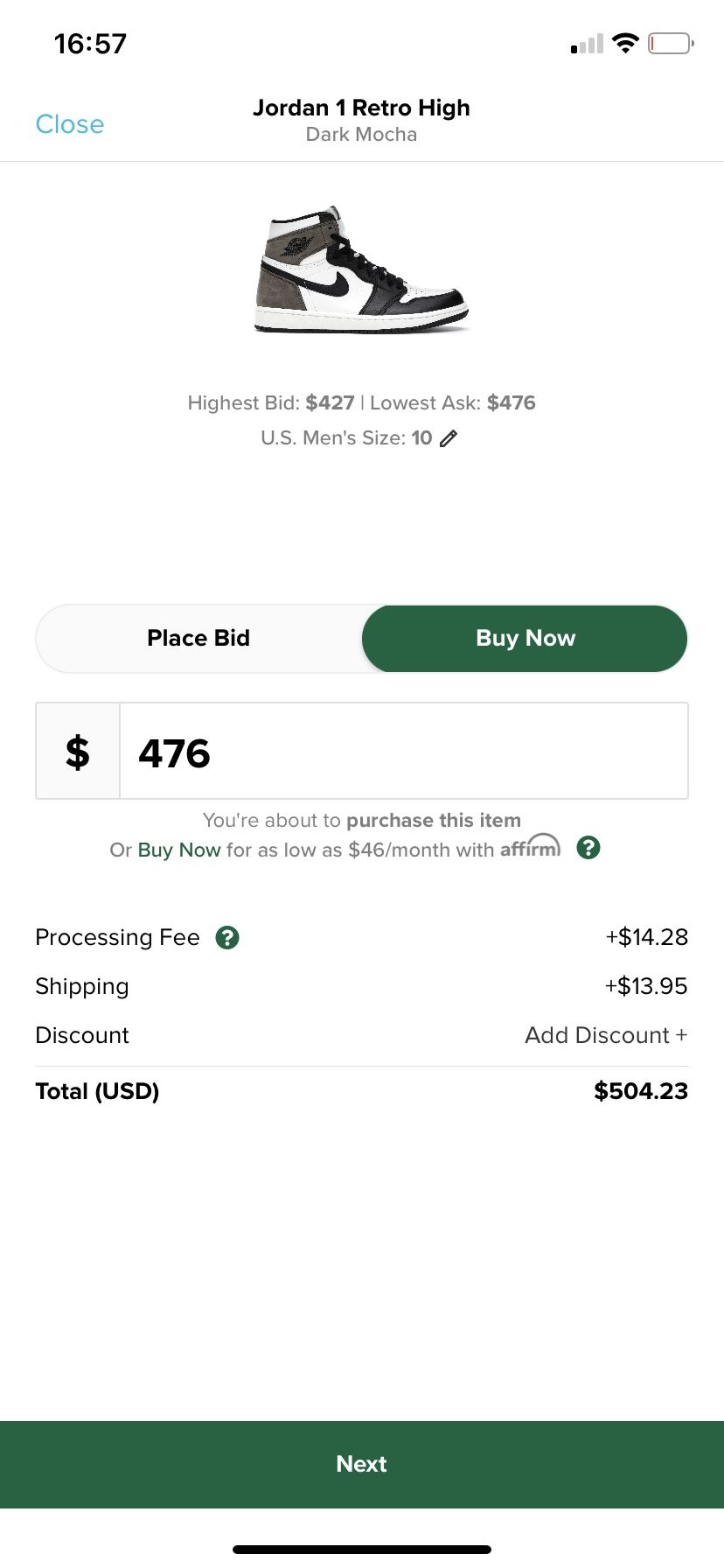This image showcases a screenshot from a tablet device displaying an online purchase interface for the Jordan 1 Retro High Dark Mocha sneakers. In the top-left corner, the time reads 16:57, while the top-right corner indicates a nearly empty battery, a full Wi-Fi signal, and a somewhat weak telephone signal. Below this status bar, the focus is on the sneaker purchase details.

At the forefront, there's a prominently elongated image of the sneaker, featuring a distinctive Nike swoosh. The sneaker sports a black and white color scheme, with white sides, black accents on the heel, over the laces, around the toe, and a white sole with a black bottom. The interface indicates the highest bid at $427 and the lowest ask at $476 for a US men's size 10. Next to these price points is a pencil icon, resembling an eraser.

Options to "Place Bid" or "Buy Now" are presented, with the lowest ask price of $476 displayed in bold black letters. The interface informs that the user can buy the item outright for the same price, or alternatively, opt for monthly payments starting at $46 through Affirm. Affirm is highlighted in green, accompanied by a curved icon above it and a green circle with a white question mark to its right.

Additional cost details include a processing fee of $14.28 and shipping costs of $13.95. A discount can be applied by clicking on a plus sign. The cumulative total is stated clearly in USD at $504.23.

At the bottom of the screen, a green banner spans across the entire width with the word "Next" in white letters, inviting the user to proceed with the transaction.